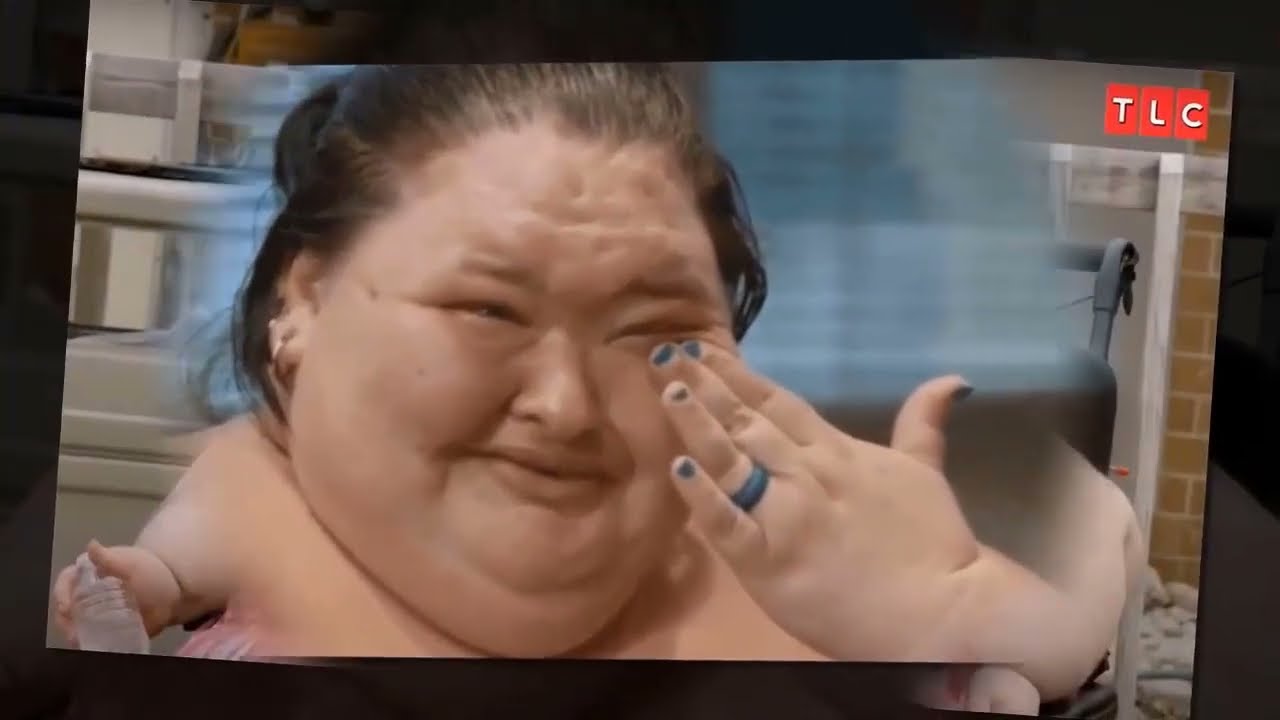The image is a detailed screenshot of the TV show "Thousand Pound Sisters" airing on TLC. It features an overweight white woman who is crying and wiping her tears with her left hand, which is adorned with blue nail polish and a blue ring on her ring finger. She has short black hair styled in a ponytail. The TLC logo, consisting of three small red boxes with white letters, is prominently displayed in the upper right corner of the screenshot. The background is blurred, revealing some blinds, and the woman appears to be holding a water bottle in her left hand.